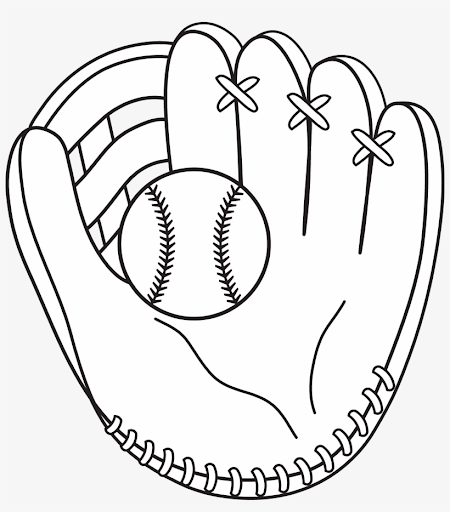This detailed black and white line drawing features a baseball mitt with a baseball nestled within its palm. The mitt is positioned with the thumb on the left and the four fingers on the right, securely held together with visible leather stitches. The open bottom of the mitt reveals additional stitching that follows the curve of the glove, emphasizing its hand-stitched construction. Between the thumb and the index finger, there's a patch where the glove catches the ball, adorned with horizontal and vertical lines enhancing its texture.

The palm of the mitt has delicate wavy black lines extending toward the left and right, converging near the centered baseball. This perfect round ball is small relative to the mitt and positioned close to the curve formed between the thumb and the index finger. The baseball itself features distinct seams characterized by curved lines with small hatch marks, mimicking the traditional stitching found on a real baseball. The background of the image is a very light gray, further highlighting the detailed and intricate design of the mitt and ball.